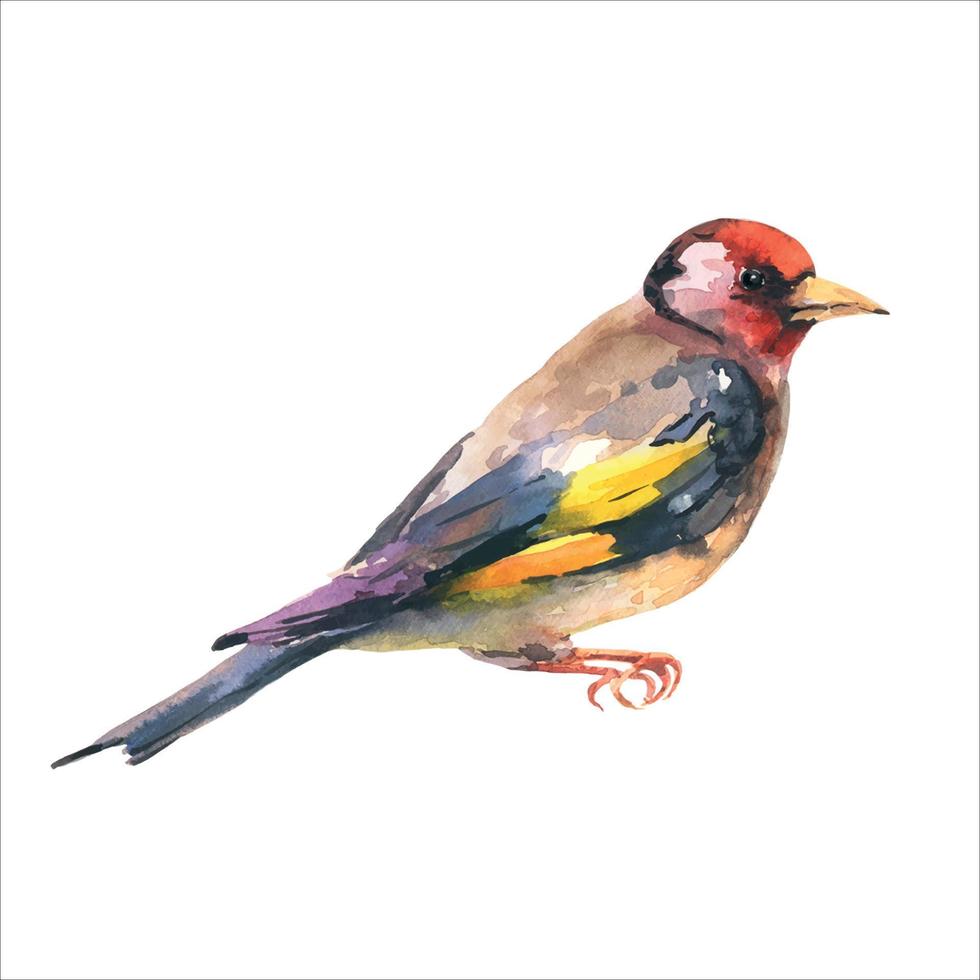This watercolor painting, presented in a square format with a thin black outline, captures a goldfinch in profile, oriented diagonally from the top right to the bottom left against a white, background-free canvas. The bird, depicted in rich detail, features a distinct red head with a yellowish beak. Its small to medium-sized body showcases a blend of colors: a cream-colored chest, a light brown belly, and an intricate array of hues on its wings and tail. The wings, folded back, transition from dark blue near the shoulders to yellow in the middle, and then to purple at the edges. The tail feathers extend gracefully, exhibiting a mix of grayish-blue and purplish shades. The orange, slightly curved claws of the bird lend to its realistic posture as if perched on an invisible branch, emphasizing the ethereal quality of the painting. The bird's eye is captured in black, contrasting subtly with the pinkish hues around its cheek area, cementing the watercolor painting's representational style.